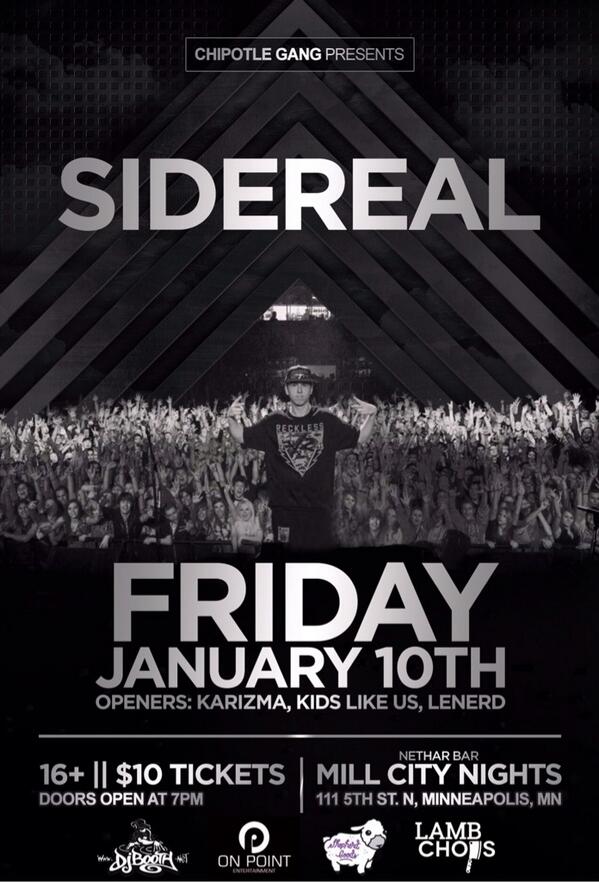The concert advertisement is predominantly black and white, with "Chipotle Gang Presents" in silver font at the top. Below that, in bold, all-caps letters, it announces "Side Reel" (stylized as R-E-A-L). The central image features a man, presumably Side Reel, on stage with a very excited crowd behind him, many raising their arms in the air. Below the image, large text declares "Friday, January 10th," followed by the openers listed as "Charisma, Kids Like Us, Le Nerd." In the bottom left corner, details state "16+, $10 tickets, doors open at 7 PM." The event location is provided on the right side: "Nether Bar, Mill City Nights, 111 5th Street, North Minneapolis, Minnesota." At the poster's base, four sponsors are displayed: DJ Booth, On Point, Shepherd (with a lamb icon), and Lamb Chops (with a unique 'P' shaped like a large chopping knife).